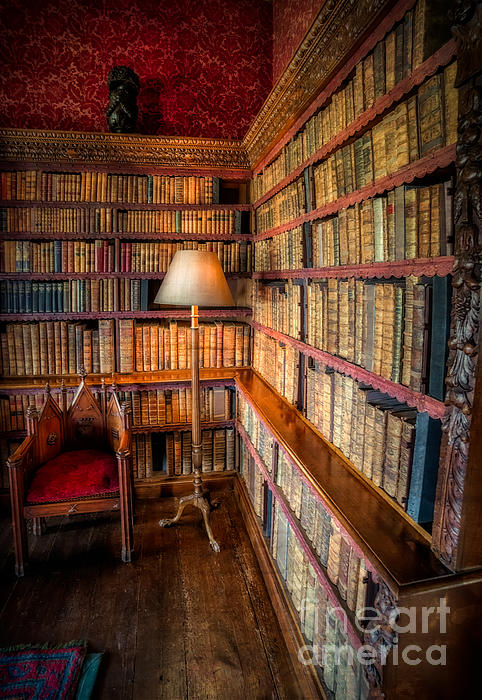The image depicts an antique library corner adorned with intricate red and yellow wallpaper featuring a light pink paisley design. Dominating the scene is a grand bookshelf crafted from gold-tinted wood with some faded red shelves, filled with old, thick brown-bound books that resemble encyclopedias. A striking detail is the gold engraved trimming at the top of the bookshelf. On top of this shelf near the back wall stands a mysterious black cylinder statue with intricate carvings. Towards the foreground, there is a small, throne-like wooden chair with a plush red velvet cushion and a crown-mimicking backrest featuring three or four pointed wooden peaks. Adjacent to the chair stands a tall, three-legged brown metal lamp with a light beige lampshade. The room's floor is covered in rustic dark brown wood, partially overlayed by a green, red, and blue rug with turquoise designs. In the bottom right corner, the text "Fine Art America" is subtly visible.